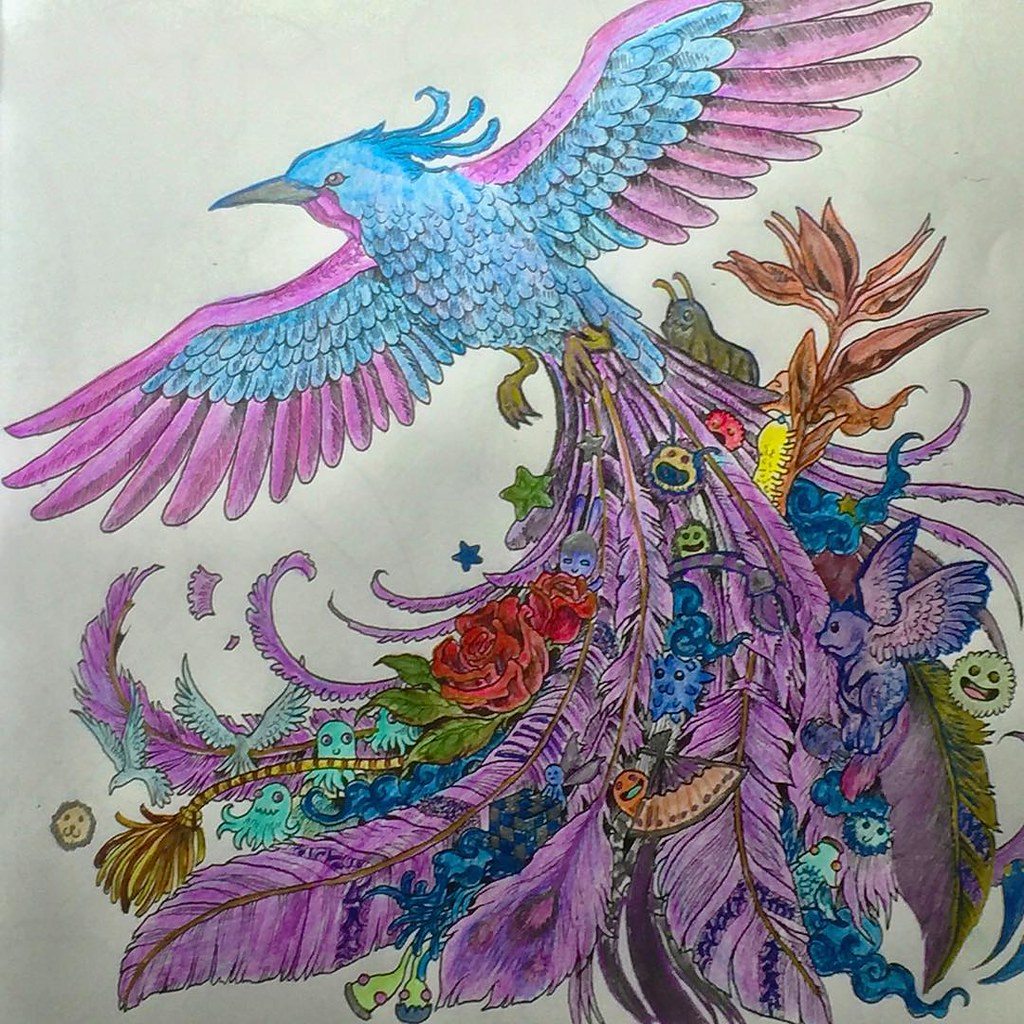This striking colored pencil drawing captures a vibrant phoenix, its body adorned with brilliant blue feathers that seamlessly transition into purple at the wingtips and tail. The enigmatic phoenix springs to life against a backdrop of intricate detailing. Unseen, the artist's signature is absent, leaving the viewer's imagination to wonder about the creator. Emerging from the phoenix’s elaborate tail feathers are miniature scenes bursting with life: two vivid red roses in full bloom, a cheerful caterpillar with a wide smile, and an enchanting purple-winged griffin. Each element is carefully interwoven into the feathers, adding layers of mystery and fantasy to this captivating piece of artwork.